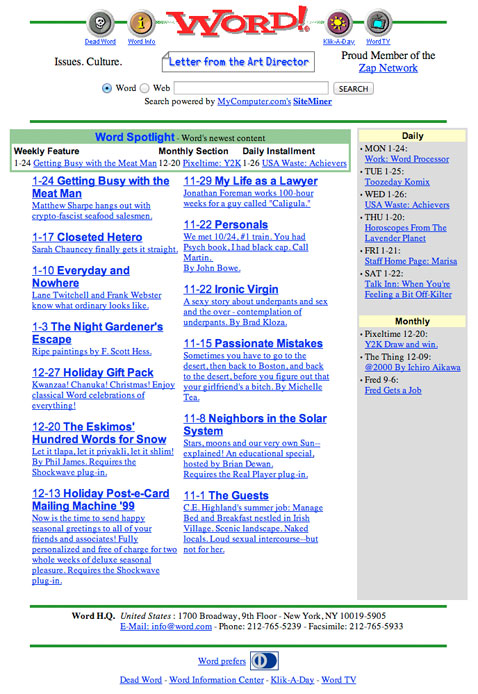This is a detailed screenshot of an old Yahoo webpage, specifically featuring a section dedicated to "Word." The word "Word" appears prominently in red at the top center of the webpage. To the left of "Word," there are two icons: one labeled "Dead Word" and the other "Word Info." To the right, there are additional icons labeled "Kill a Day" and "Word TV."

Directly beneath the "Word" header is a blue banner that reads "Letter from the Art Director." Below this banner, there are two bubbles labeled "Word" and "Web," along with a search bar equipped with a search button.

On the main portion of the webpage, there is a green box at the top with the text "Word Spotlight: Newest Words, Newest Content." Below this box, the content is organized into two columns, each with blue underlined titles and corresponding descriptions. The first column's header reads "I 124: Getting Busy with the Meat Man."

On the far right side of the page, there is a gray box divided into two sections—"Daily" at the top and "Monthly" at the bottom. Each section contains links along with dates and days.

At the bottom of the page, there are two green borders enclosing contact information. The text within these borders includes:
- "Word HQ, United States, 1700 Broadway, 9th floor, New York, NY 10019-2590"
- An email hyperlink: "info@word.com"
- Phone number: "(212) 765-5239"
- Facsimile: "(212) 765-5933"

Additionally, there are several links at the bottom, starting with "Word Prefers" which is accompanied by an icon resembling a payment processor. Other links include "Dead Word," "Word Information Center," "Click a Day," and "Word TV."